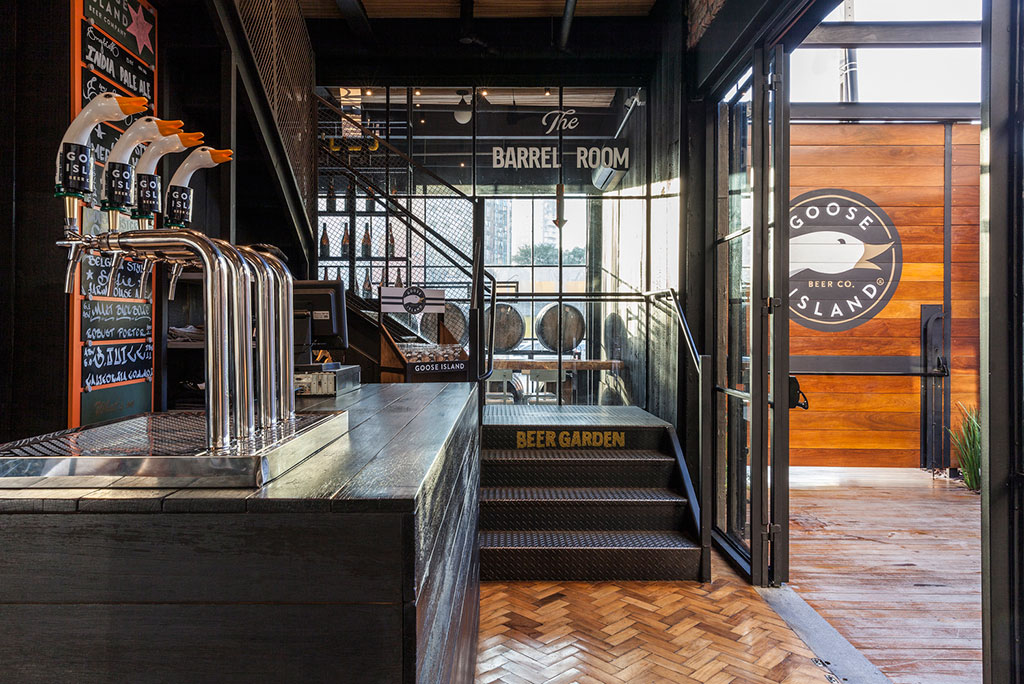The photograph depicts the interior of a Goose Island Beer Company establishment, which combines elements of a restaurant, bar, and brewery. The entryway is adorned with light wood and a prominently displayed sign featuring a white goose with an orange beak, labeled "Goose Island Beer Company." The flooring varies between cobblestone and parquet wood, leading to a staircase marked "Beer Garden," hinting at an outdoor drinking area. Above the staircase, a sign reads "The Barrel Room," indicating an indoor space within the bar. 

On the left, the photograph captures a bar area with distinctive beer taps shaped like goose heads, each labeled "Goose Island." Behind the bar, a large blackboard with orange trim showcases drink options, although the text is not fully legible. The space also includes open doors leading to an outdoor area with cedar slats and a circular black logo with a goose head, reiterating the Goose Island brand. The blend of indoor and outdoor elements, along with the specialized décor, strongly suggests the establishment functions as a brewery and a beer garden, offering a unique and cohesive drinking experience.